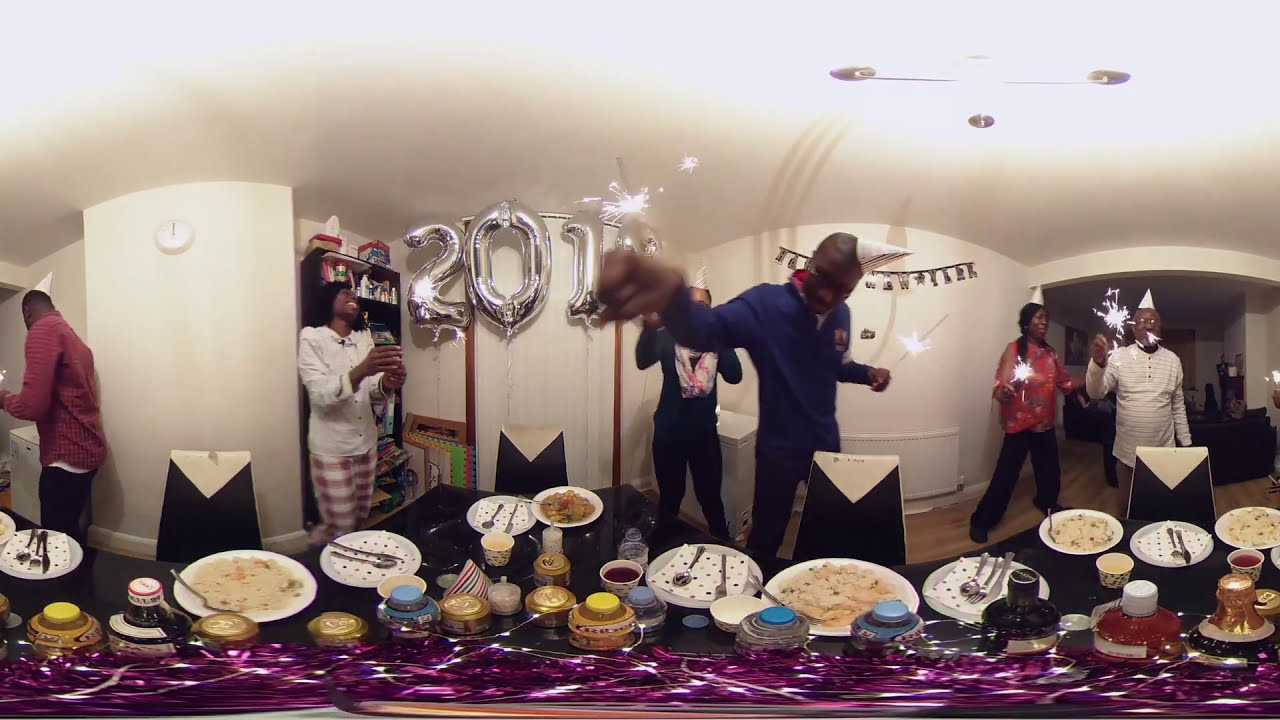This panoramic image captures a lively New Year celebration in a white-walled room adorned with a "2018" balloon on the far left. The white ceiling and light brown wooden flooring create a bright and welcoming atmosphere. At the forefront is a table draped in a black tablecloth and decorated with shiny purple garland. The table is laden with plates of food, including fried rice and other entrées, alongside colorful jars and bottles in hues of yellow, blue, and red. White polka-dot napkins, forks, and knives are neatly arranged across the plates.

Surrounding the table are square-shaped chairs with white headrests and black upholstery. Six celebrants, composed of four men and two women, stand behind the table, each holding a sparkling sparkler. They are festively dressed with cone-shaped white hats. One woman is visibly laughing, while another man is caught in mid-gesture. The room is brightened by the joy and energy of the New Year celebration, captured in this dynamic and detailed moment.